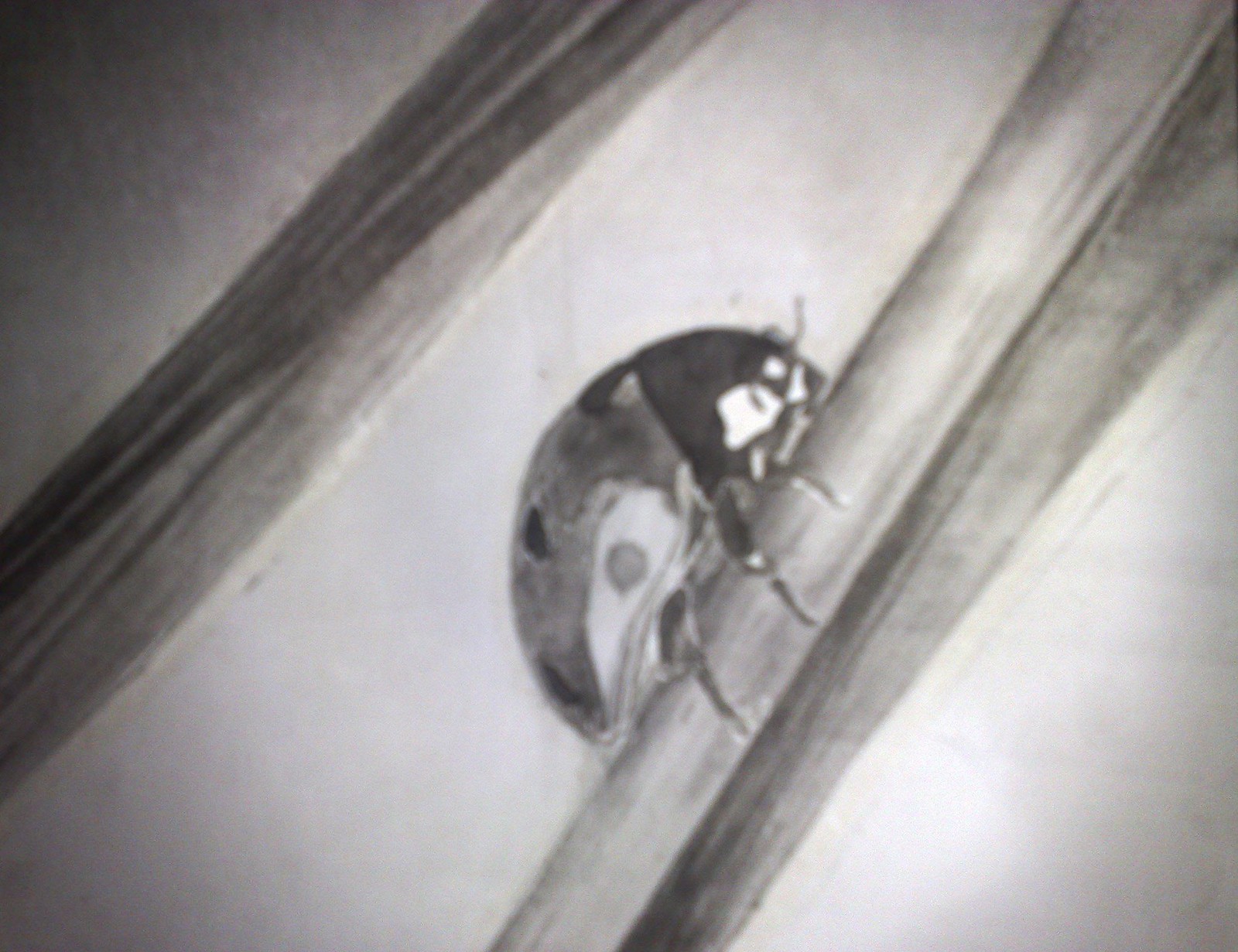This black-and-white photograph captures an intimate, up-close view of a ladybug meticulously crawling along the stem of a plant. The detailed image highlights one of the ladybug's eyes and its delicate feelers, providing a rare glimpse into its facial features. The ladybug's legs are clearly visible as they grip the plant stem, demonstrating its intricate anatomy and the texture of the stem itself. The insect's back legs exhibit a lighter coloration compared to the rest of its body, adding a subtle contrast to the composition. Above the ladybug, there is a darker plant stem that gradually lightens towards the bottom, creating a nuanced background. Despite a slight streaking effect and faint lines across the image, the overall quality remains impressive, allowing the viewer to appreciate the finer details of this tiny creature's journey.